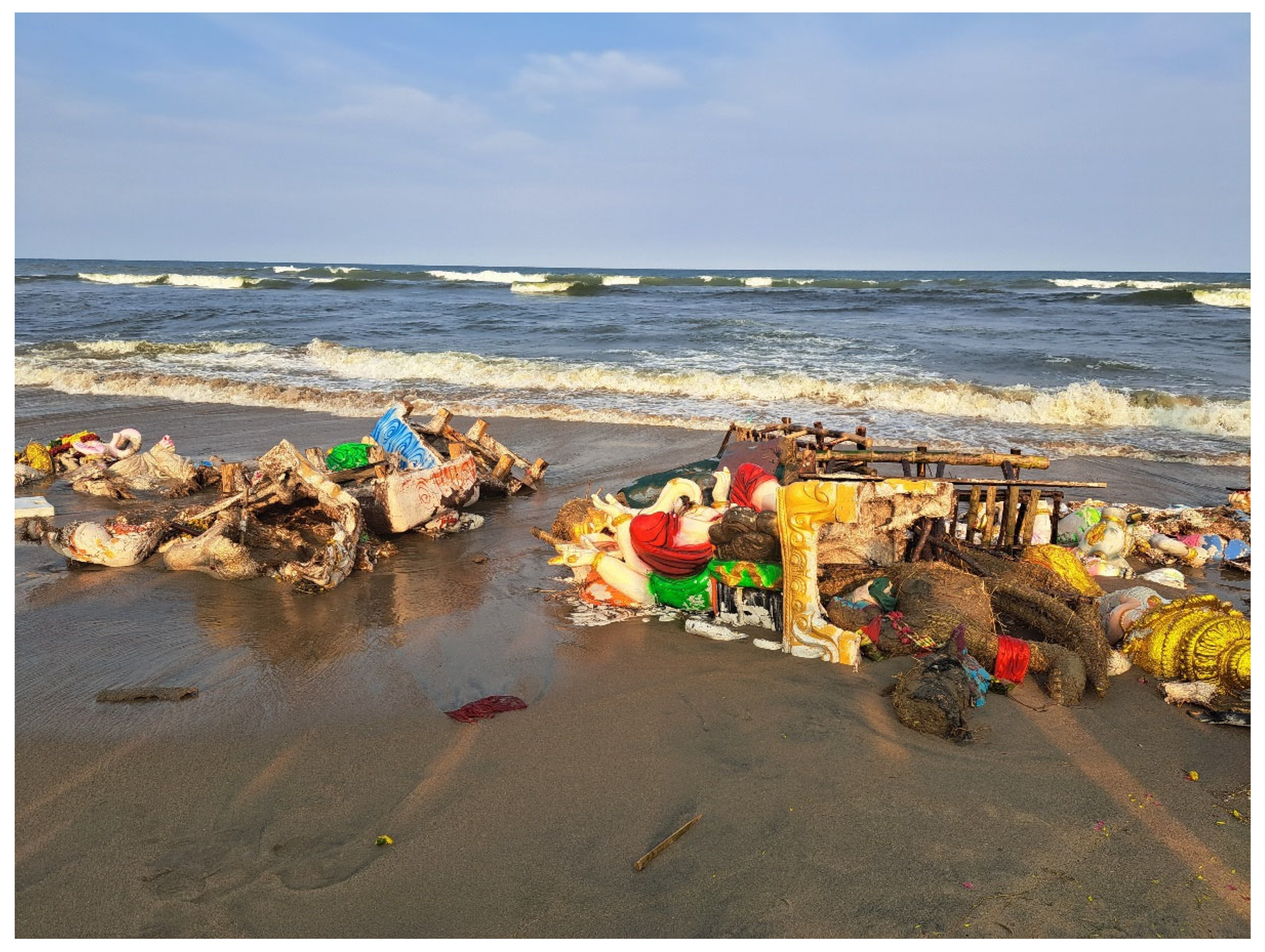This photograph captures a beach scene from the perspective of someone standing close to the water's edge, looking towards the horizon. The top quarter of the image is a light blue sky punctuated with streaky white clouds, suggesting a clear day with plenty of light, though no sun is visible. Below, gentle waves from the ocean break towards the shore, leaving a film of water where they meet the dark brown, wet sand. The most striking feature is the extensive array of trash strewn across the beach, forming several clusters. In the foreground, the left and right sides of the image are dominated by large patches of discarded items, which include a variety of objects such as pieces of furniture, toys, and household items, all appearing old, dirty, and wet, some even covered in seaweed. The central part of the beach features a path leading towards the water, flanked by these refuse piles. The colorful debris, marked by yellows, reds, greens, and blues, creates a stark contrast to the natural landscape. The scene evokes a sense of neglect and pollution amidst the natural beauty of the beach.